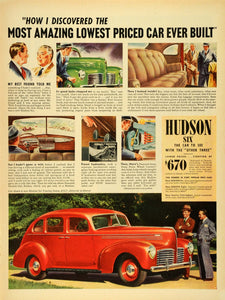This image showcases a yellowed, vintage magazine advertisement for the Hudson Six, priced at $670. At the top of the vertically rectangular page, bold black text on a light beige background reads, "How I discovered the most amazing lowest priced car ever built." Below this headline are three illustrations in a row: one of two men in suits talking, another of a man in a dark gray suit and a white and black hat inspecting a green car from the 1940s or 50s, and a final image of the men examining the car's spacious back seat. Each illustration is accompanied by a paragraph of black text beneath it.

In the middle section, three more images are displayed in a row: the man in the gray suit driving the car from an interior view, an image of the gas pedals with the man pointing at them, and a third, less discernible picture. Below these images are additional descriptive text paragraphs.

On the right side of this middle section is a darker beige rectangular area filled with black text, including mentions of the Hudson Six and its price at $670. At the bottom of the page, a large photograph depicts a vintage red car pointing to the right, with two men in suits standing in front of it. The background subtly includes trees and a hint of grass, indicating an outdoor setting.